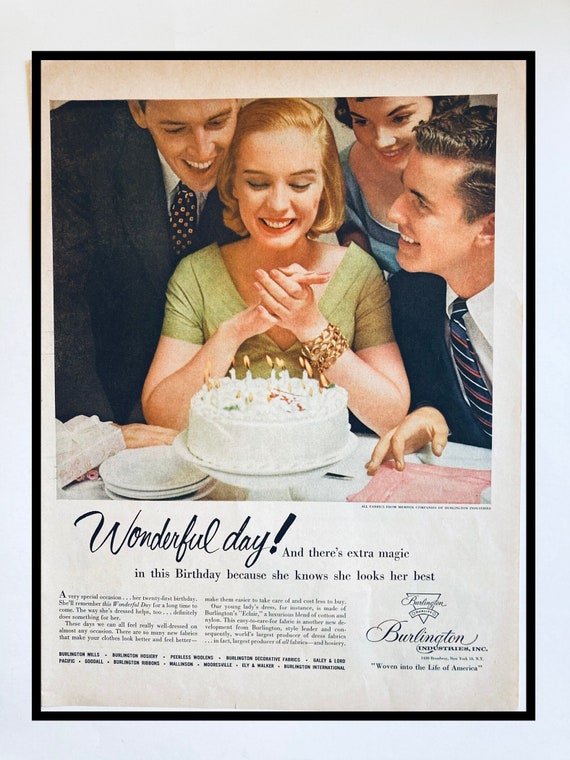This circa late 1950s to early 1960s photograph, likely a magazine advertisement, is bordered by a grayish-blue frame with black on the outside and white on the inside, set against a white background. The ad features a young woman in her mid-twenties, adorned in a green dress with short sleeves, and a gold bracelet on her left wrist. Seated at a table, she clasps her hands in front of her smiling face, gazing at a white cake with lit candles. Surrounding her are two men in suits, complete with white shirts and ties, each standing on either side of her shoulders. To the right, slightly behind the man, stands another woman with short black hair, dressed in a greenish-blue dress, also smiling at the cake. Below the image, in black script, reads "Wonderful day!" followed by, "There is extra magic in this birthday because she knows she looks her best." Further text in two paragraphs appears below, with "Burlington Industries, Inc. woven into the life of America" on the right.